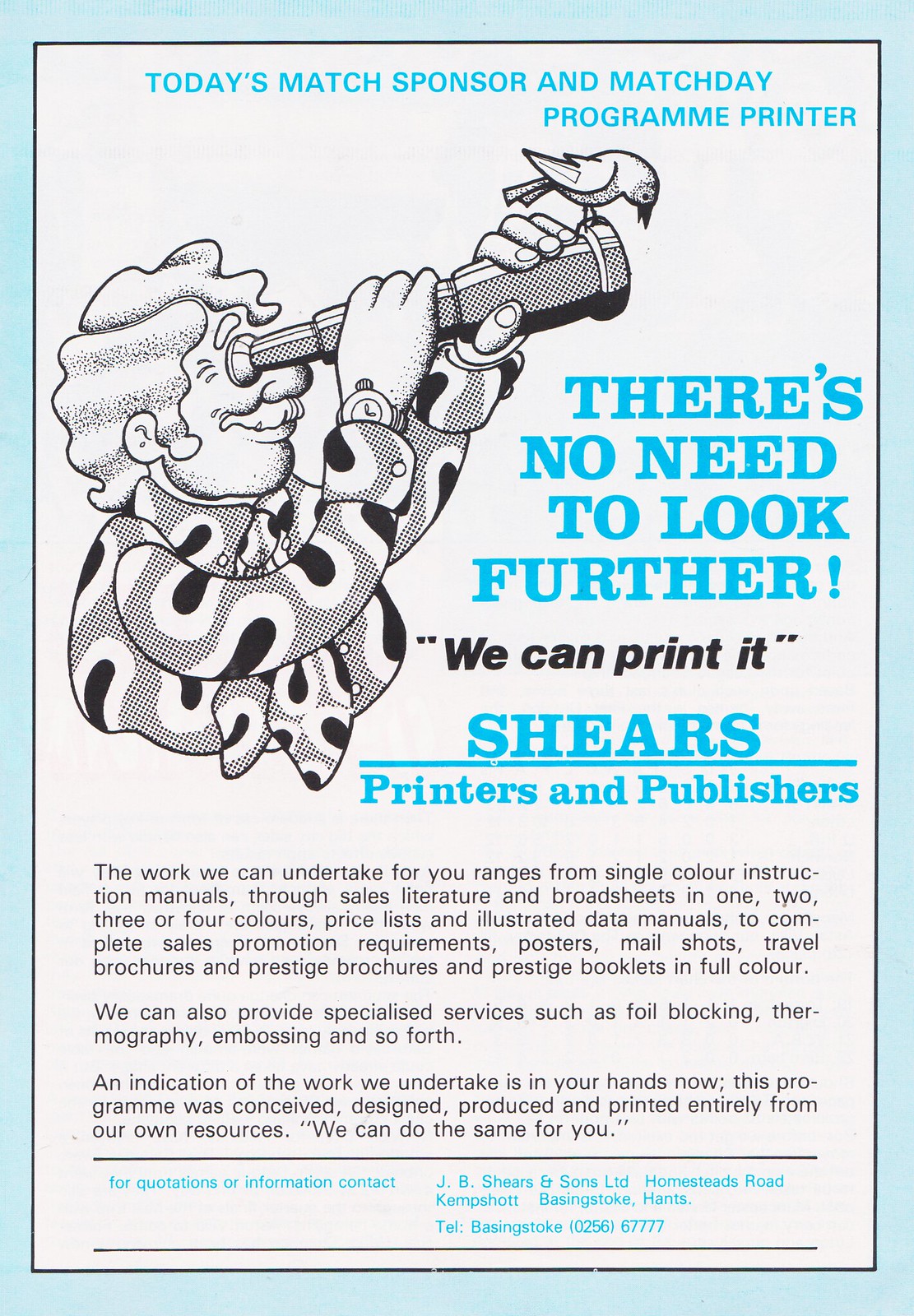This vibrant flyer for Shears Printers and Publishers, primarily in white with a baby blue border, prominently features a detailed cartoon illustration of a cheerful man. He is dressed in a textured, patterned jacket and matching tie, holding a spotting scope with a bird perched at the end, peering back at him. The advertisement proudly announces Shears as today's top match sponsor and Match Day program printer with the encouraging slogan, "There's no need to look further. We can print it." Following this, in black lettering, the flyer elaborates on the extensive range of printing services Shears offers, including single-color instruction manuals, multi-color sales literature, illustrated data manuals, comprehensive sales promotions, posters, mail shots, travel brochures, and prestige booklets. The comprehensive services are underscored by the company's flexibility in handling projects across one to four colors. At the bottom, in baby blue text, additional service details and contact information are provided, highlighting Shears' commitment to quality and customer satisfaction.